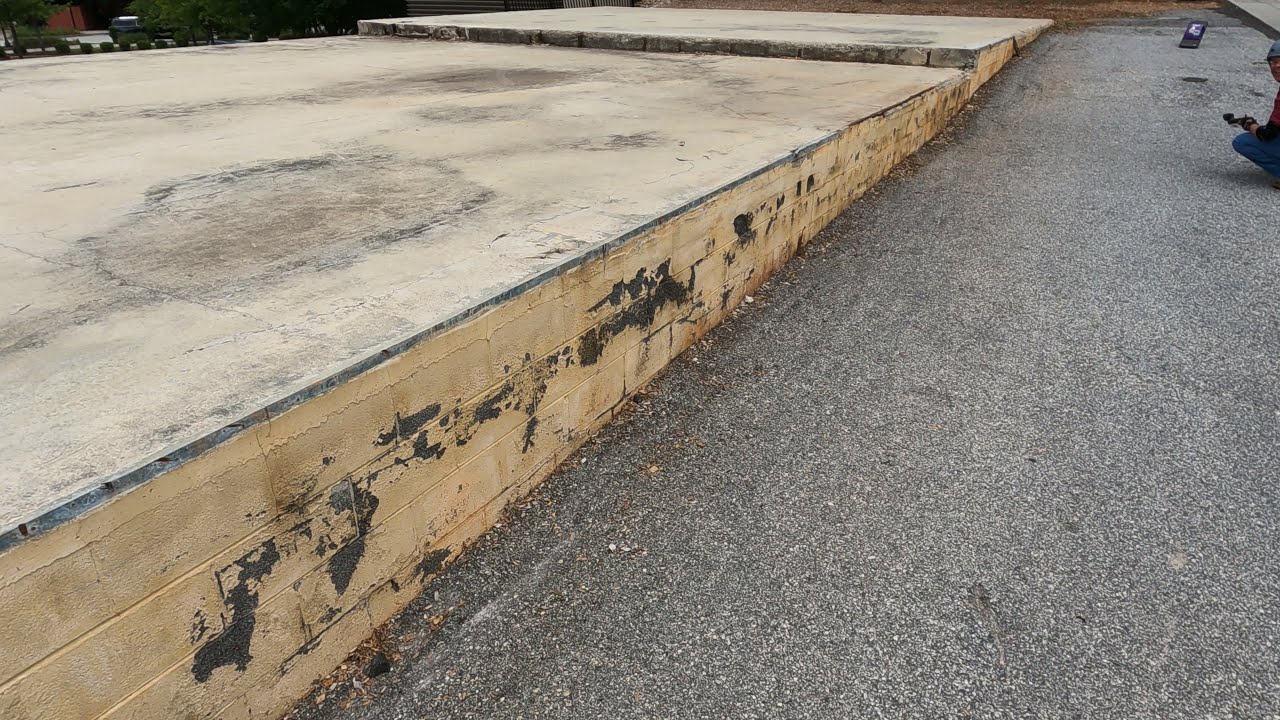The photograph captures an outdoor scene, primarily focusing on the ground. Central to the composition is a distinct gravel or concrete path, gray in color, that traverses horizontally across the frame. To the left of this path, there is an elevated surface constructed from yellowish-orange bricks, forming a wall-like structure. The structure is marked with several dark gray and black smudges, likely caused by paint, weather, or age, lending a worn appearance to the bricks. In the upper right corner of the image, a man, partially cut off, is seen crouching down, apparently holding a camera and positioned in front of what seems to be a laptop. This photo is well-lit, indicative of being taken outdoors during the daytime, with ample natural light providing clear visibility of the details.